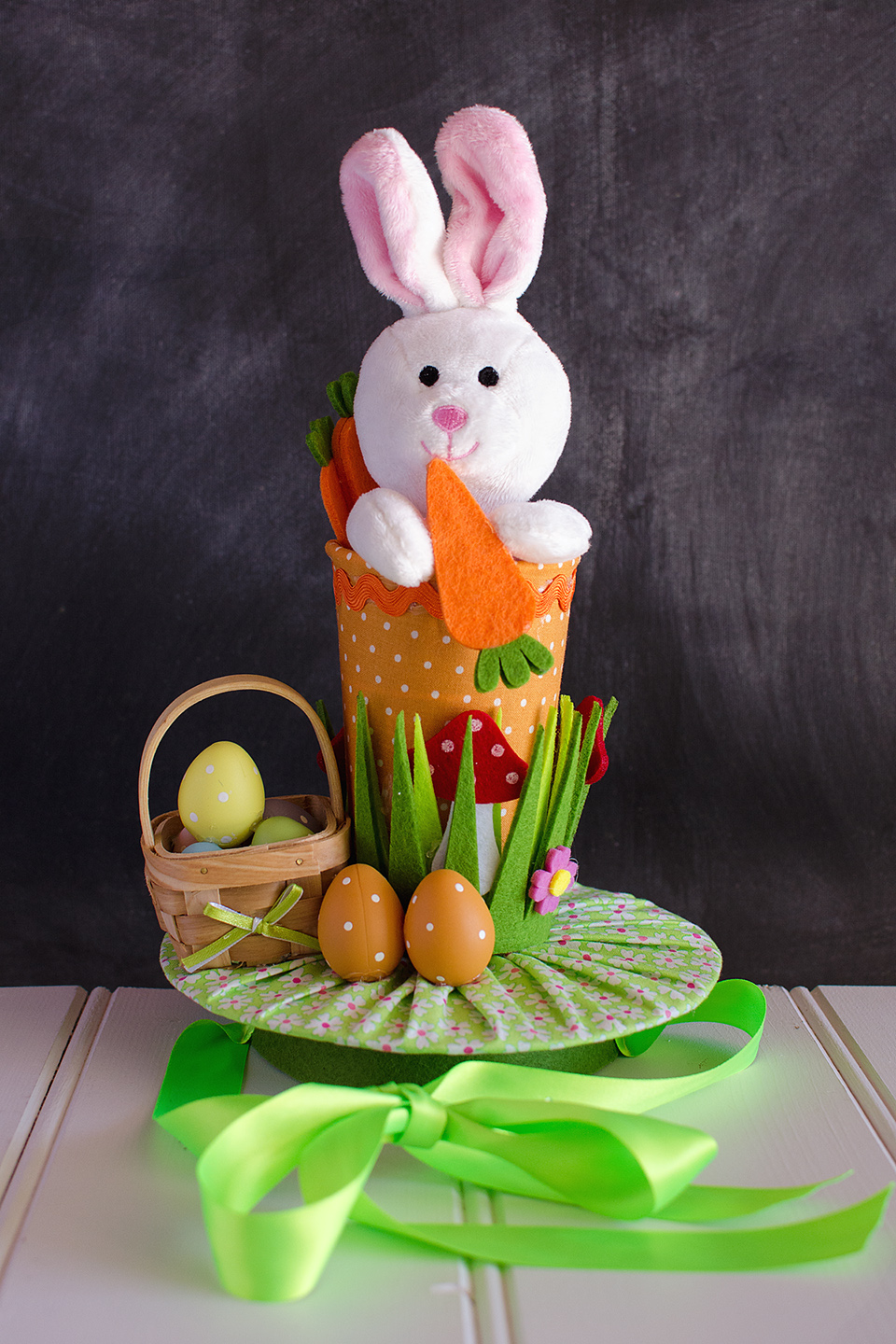The image depicts a detailed Easter-themed decoration featuring a plush pink rabbit with long ears that have white edges and pink insides. The rabbit, adorned with a cheerful smile and black eyes, is nestled inside an orange, white-spotted, conical felt container resembling an upside-down hat. This container sits atop a round base covered in green cloth with pinkish stars and edged with a large green ribbon in the foreground. The rabbit holds an orange felt carrot and is accompanied by two or three similar felt carrots placed behind it to the left.

Surrounding this central figure is additional festive decor: at the base in front, there are several brown eggs with white dots, while to the left, a small wooden Easter basket contains multiple eggs, including a prominent yellow egg with white dots on top. Attached to the base, we see sharp felt triangles mimicking grass and a pair of decorative red-capped toadstools. The entire setup rests on what appears to be a white striped wooden surface, with a blackboard-like background, giving the impression of a classroom setting.